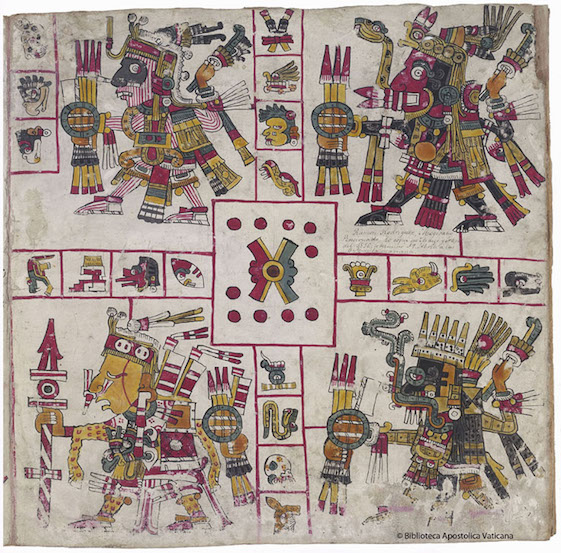This intricate illustration, likely created with pen and ink and housed in the Biblioteca Apostolica Vaticana in Italy, features a layout divided into four sections by a central cross. Each quadrant depicts a highly detailed figure, possibly representing indigenous warriors from Aztec or Incan cultures, adorned with elaborate headdresses and wielding various weapons such as arrows, spears, and torpedo-like objects. The figures exhibit typical indigenous stylings, with ornate decorations and colorful attire in maroon, yellow, light gray, and dusty pink hues. At the intersection of the cross, there is a central, larger rectangular shape filled with more intricate images, surrounded by smaller sections of similarly decorated motifs. The background is subtly shaded with faded colors, adding to the complexity and beauty of the artwork.